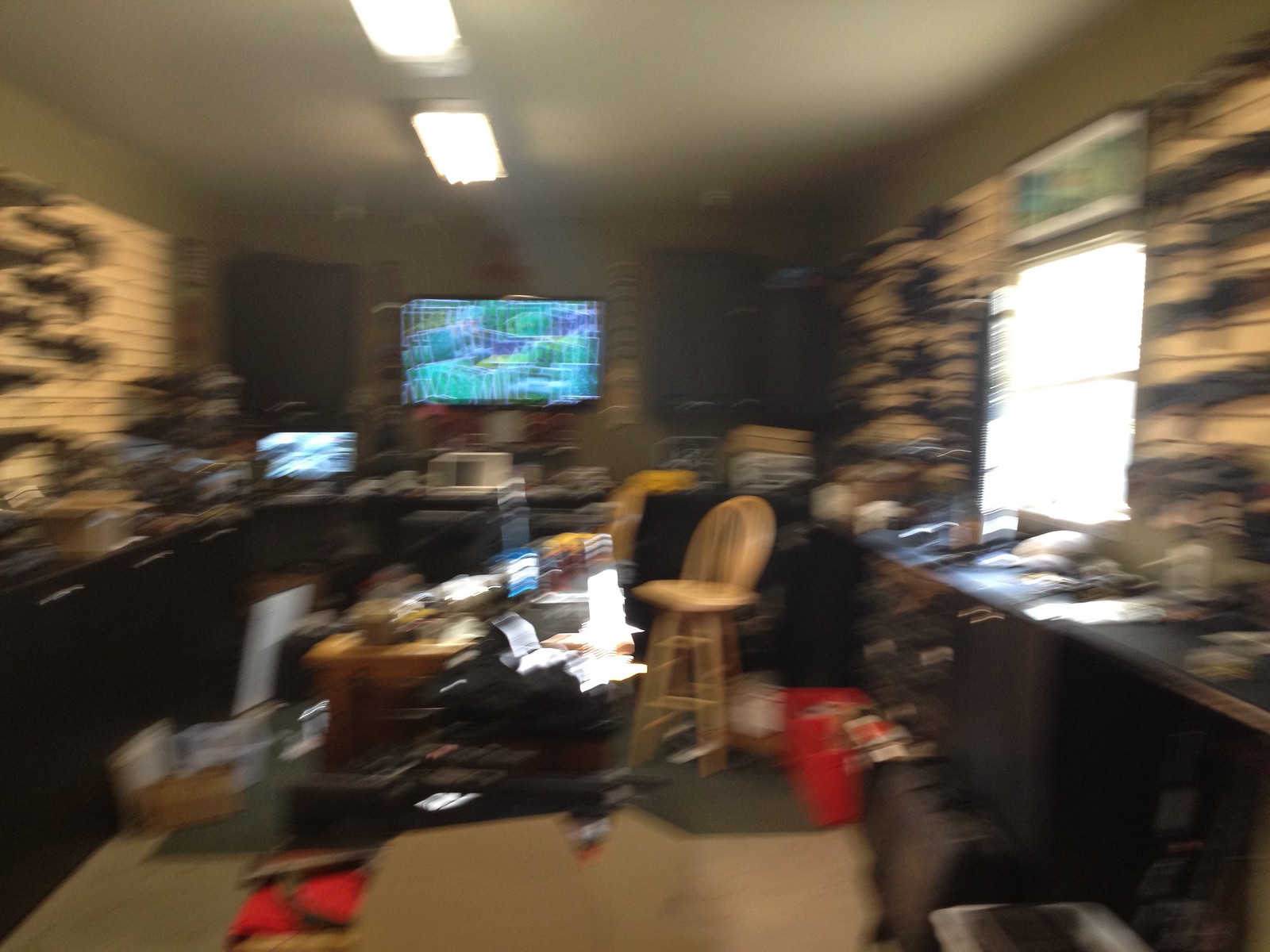In this slightly blurry photograph, the interior of a gun shop is captured in detail. Dark-colored cabinetry lines the walls, providing a stark contrast to a light-colored wooden chair that is slightly elevated in the foreground. Arrayed around the shop are several black bags and numerous black plastic gun cases, contributing to the store's organized yet busy atmosphere. On the wall, a variety of predominantly black firearms are mounted on a white backdrop, adding to the visual complexity of the scene. An overhead light casts a glow, illuminating a black security monitor that displays multiple images in hues of green, yellow, and white. Additionally, a computer rests on the counter amidst an assortment of scattered objects, adding to the functional but cluttered ambiance. A window allows sunlight to filter into the room, providing a touch of natural light to the otherwise utilitarian space.